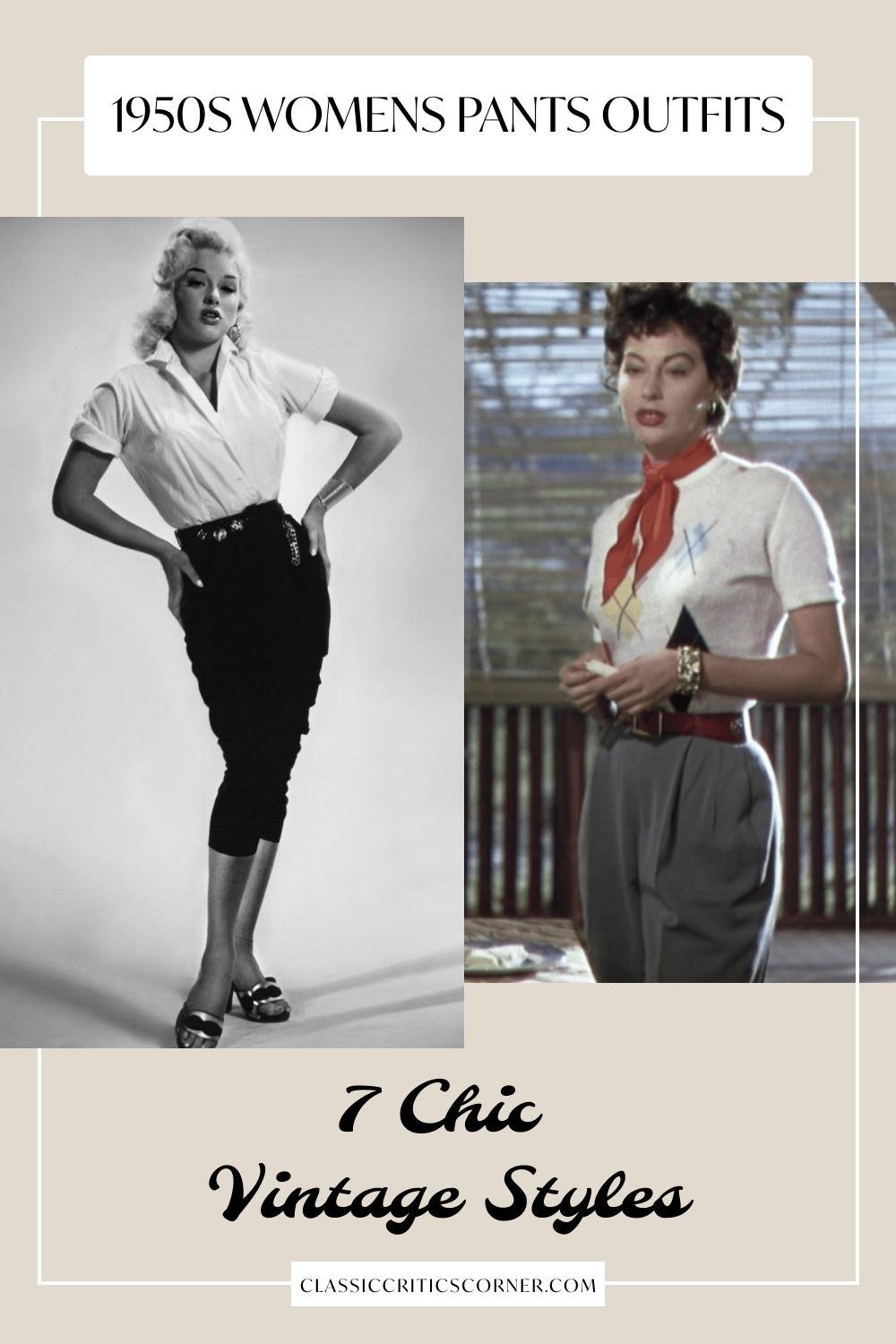Title: ClassicCritiquesCorner.com: The Worst 1950s Women's Pants Outfits

Caption: Featured on ClassicCritiquesCorner.com, this vintage photograph critiques two distinct 1950s women's pants outfits under the title "The Worst 1950s Women’s Pants Outfits." The left image, a classic black and white shot, showcases a woman reminiscent of Marilyn Monroe, wearing a short-sleeved white shirt paired with slim, cropped black pants and sandals. On the right, a color photograph depicts a woman with a red scarf around her neck, sporting a white sweater adorned with various black and blue patterns, including a yellow and blue square design and a black parallelogram. She completes her ensemble with gray pants and a brown belt. The article, titled "Seven Chic Vintage Styles," critiques these vintage looks while showcasing their potential influence on modern fashion trends.